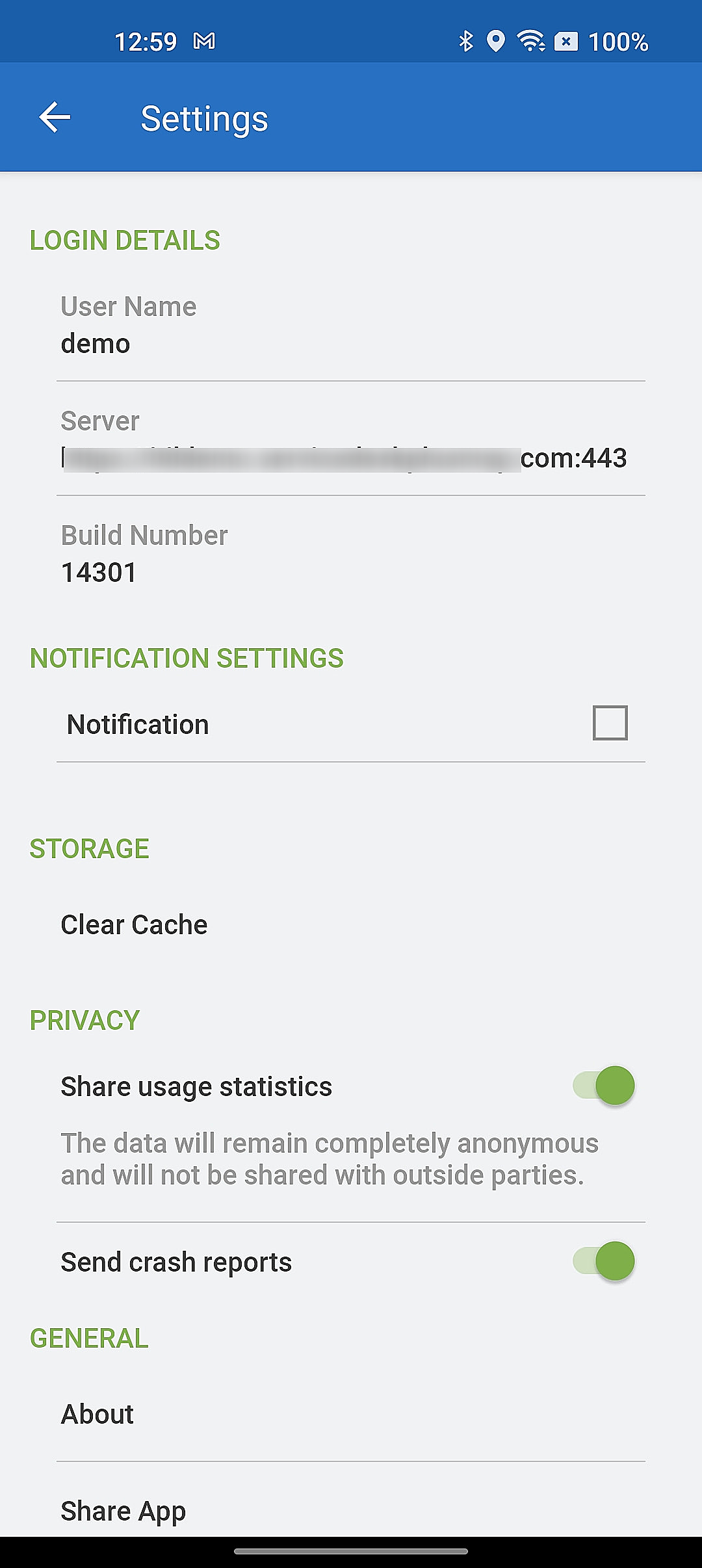The image features a frequently seen settings screen, likely from a mobile or web application. At the top left, there is a back arrow icon. Below this, the section heading, "Login Details," is displayed in green text. Under "Login Details," the username field is filled with "demo," while the server detail is blurred out. The build number "com443 build number 14301" is also in green text.

Following this, there is a section titled "Notification Settings," with "Notification" written next to a checkbox. Further down, "Green Storage" and "Clear Cache" are highlighted with bold text.

In addition, there is another section labeled "Privacy," also highlighted in green. Under privacy settings, the options "Share Usage Statistics" and "Send Crash Reports" are both turned on, indicated by green toggle buttons. 

Finally, there are additional green-highlighted categories named "General," "About," and "Share App." Beneath the "Share Usage Statistics" setting, there is some explanatory text providing more context.